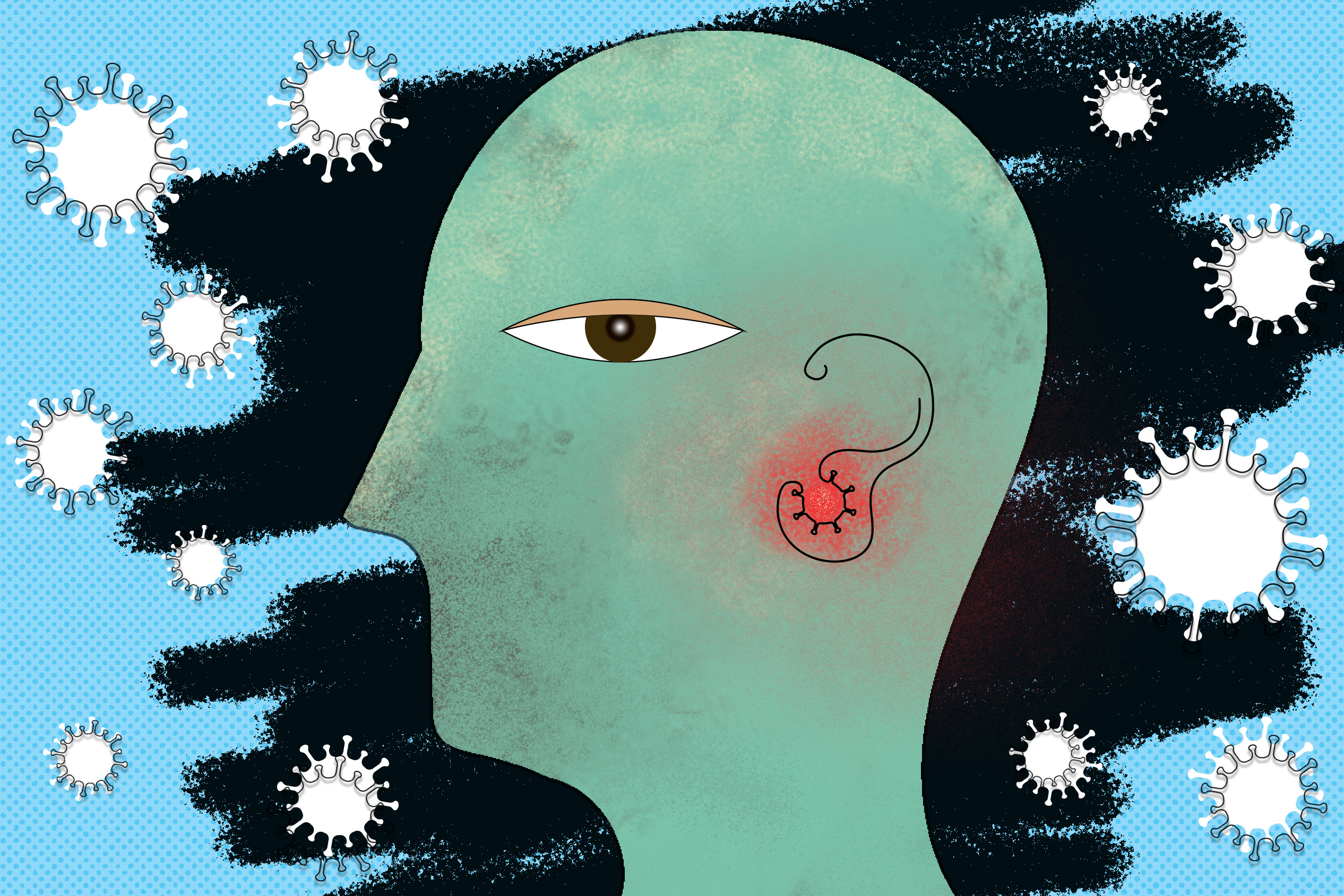This detailed, hand-drawn illustration, reminiscent of artwork found in medical journals or psychology articles, showcases a minimalist line drawing of a human head in profile, facing left. The head, colored green, features a single, prominently detailed eye with a white dot at the center, surrounded by a black circle and a brown iris, giving it a half-closed appearance. The ear is outlined with a striking black line and appears red and irritated within its contours. The background is a light blue, adorned with darker blue polka dots and chaotic, crayon-like black scratches. Encircling the head are numerous line-drawn representations of the coronavirus, distinguished by white circles with protruding spiky proteins. This emphasizes a modern, abstract style with a strong focus on intricate details, capturing a blend of contemporary artistry and scientific imagery.